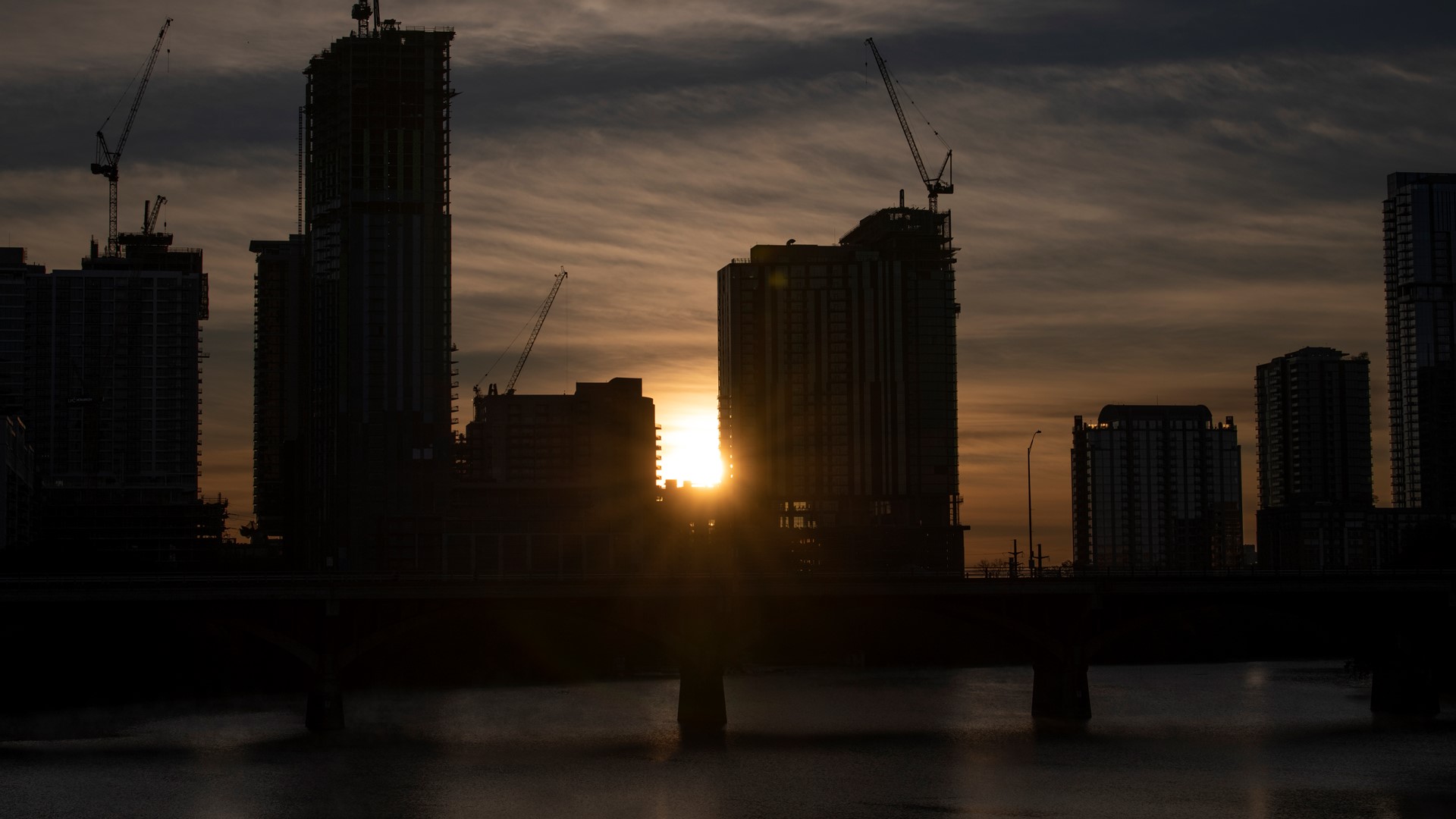This outdoor photograph captures a serene sunset scene, where the sun is positioned directly in the center of the image, partially obscured by tall skyscrapers that dominate the background. These buildings, some of which are still under construction as evidenced by cranes perched on their rooftops, are bathed in the orange and white glow of the descending sun. The sky exhibits a gradient from bright yellow near the horizon to deeper blues, adorned with long, wispy clouds. In the foreground, a dark, bridge-like structure stretches horizontally across the image, supported by five distinct pillars—two at the edges and three aligned centrally. Below the bridge lies calm, dark grayish-blue water, possibly from a river or lake. The perspective hints at an elevated or floating island setting, creating a dramatic and captivating scene.